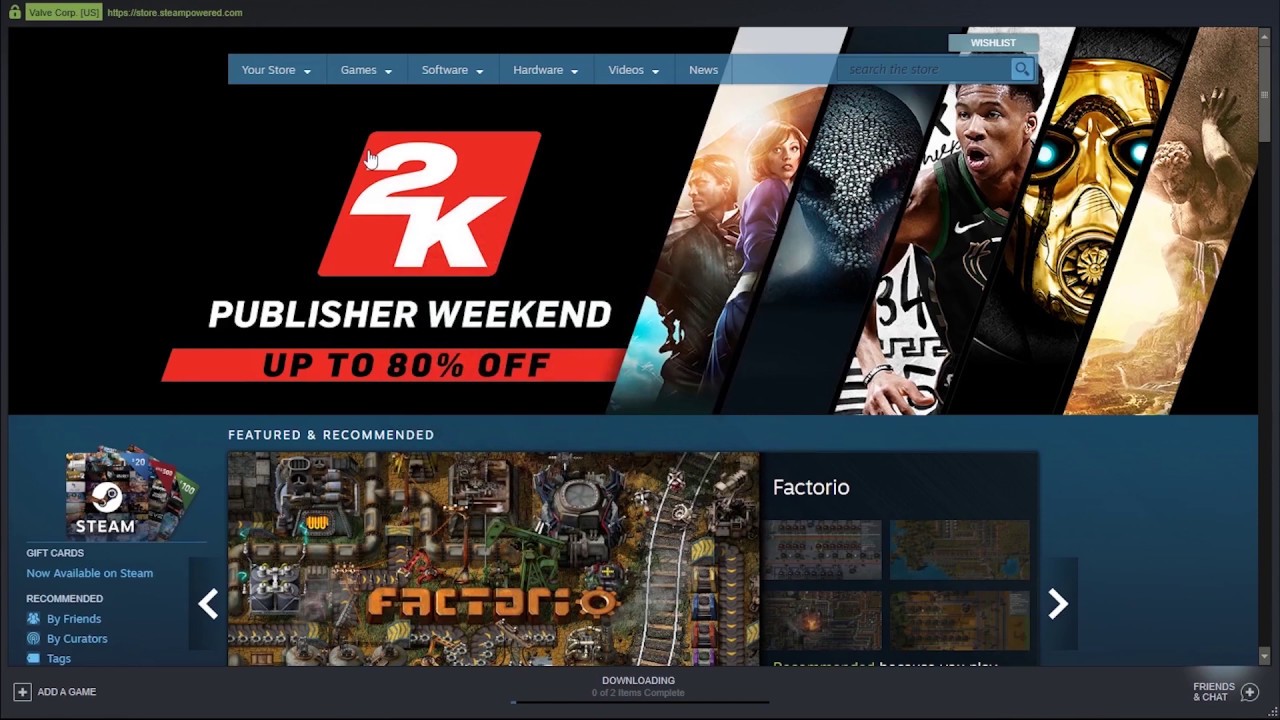The image is a promotional banner for a "2K Publisher Weekend" event, featuring discounts of up to 80%. At the top, there's a search bar followed by navigation categories labeled as Watch, Wishlist, Your Show, Games, Software, Hardware, Videos, and News. 

Central to the banner are several images representing various movies or games. One shows a man and a woman engaged in combat, another depicts an alien, and a third features a man who appears to be a basketball player. There's also an image of a person wearing a gas mask with possibly glowing blue eyes, and another portraying a deity-like figure that resembles Jesus or a god holding a statue of the world on their back.

Towards the bottom, there is a section titled "Featured and Recommended," highlighting the game "Factorio" and the gaming platform "Steam." Near the very bottom of the image, options for "Add a Game" with an accompanying plus symbol inside a square, "Downloading (0 of 2)," and "Friends and Chat" with a chat bubble containing a plus sign are displayed.